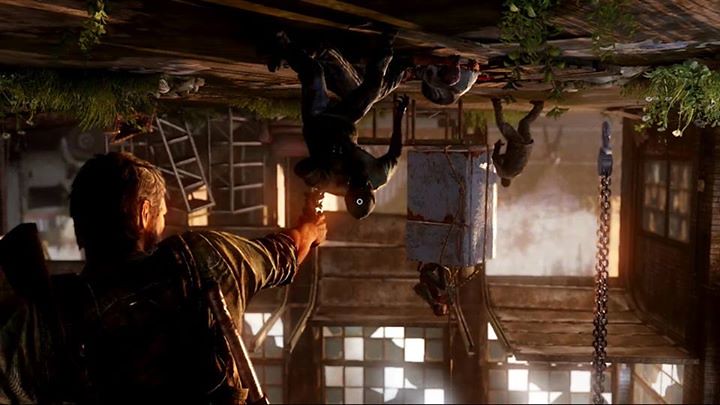In this detailed game screenshot from "The Last of Us," the image presents a dramatic scene where Joel, with short brown hair and possibly a beard, is seen hanging upside down from a hook in a dilapidated warehouse. His muscular right arm is extended, holding a pistol aimed at a zombie's head. The unique perspective shows Joel upright while the world appears upside down, making the ground look like the sky at the top of the scene. Sunlight streams through broken windows, casting light into the cluttered environment filled with debris, ladders, and industrial remnants. In the background, Ellie is perched atop a metal structure, observing the chaotic scene below. Several zombies, characterized by dark grey-brown skin and glowing circles for eyes, loom around Joel, with one nearest to him and another further back. The warehouse, bathed in daylight, captures an intense and perilous moment in the storytelling of the game.